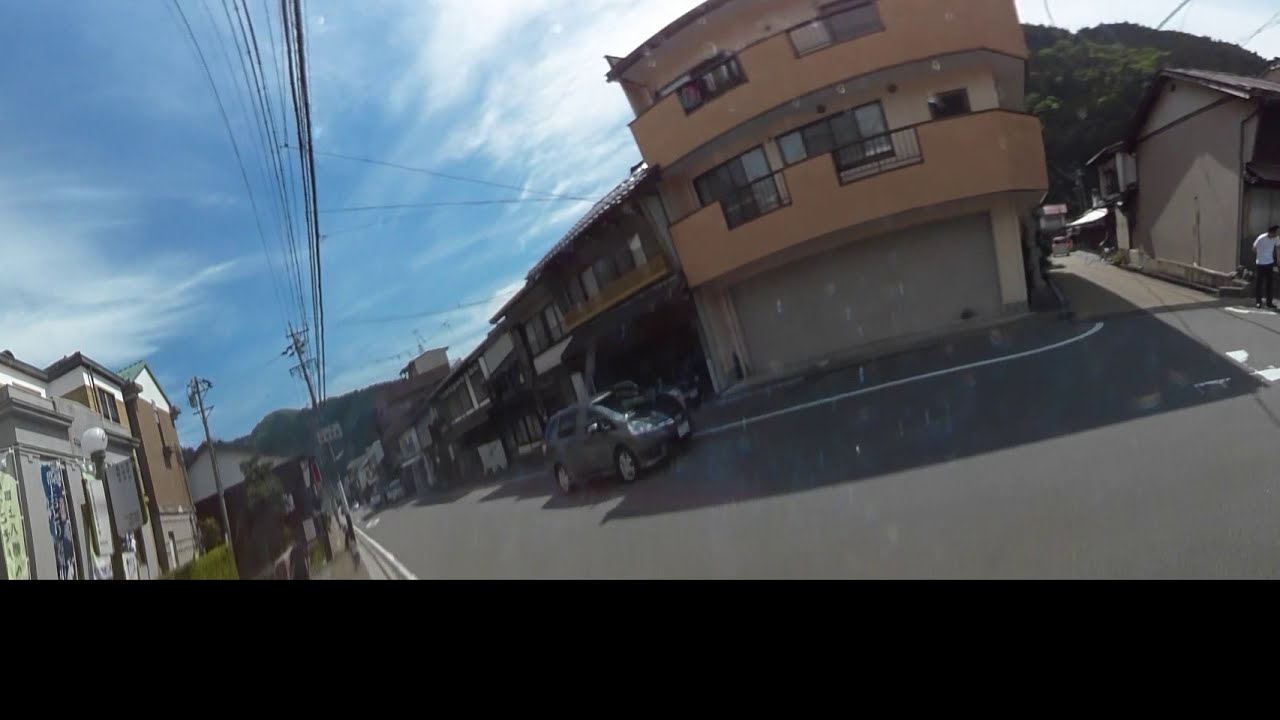The image captures a clear, daytime street view of a serene Japanese neighborhood with distinct architecture and a bright blue sky. Prominently, a three-story, rectangular residential building in tan and brown hues stands in the foreground, featuring a beige or grayish garage at the bottom and balconies on each floor. The street, lined with similar flat-roofed buildings, extends to the left and includes minimal traffic with a small car visible either driving or parked. Overhead wires are seen crisscrossing above the street, indicating a well-structured utility system. Towards the right, a person in a white shirt and black pants stands on the road, near where the sidewalks intersect. The backdrop reveals a picturesque hillside with dense trees and additional mountains faintly visible in the distance. On the right side of the brown home, an alley provides a pedestrian pathway, contributing to the neighborhood's orderly and peaceful ambiance.